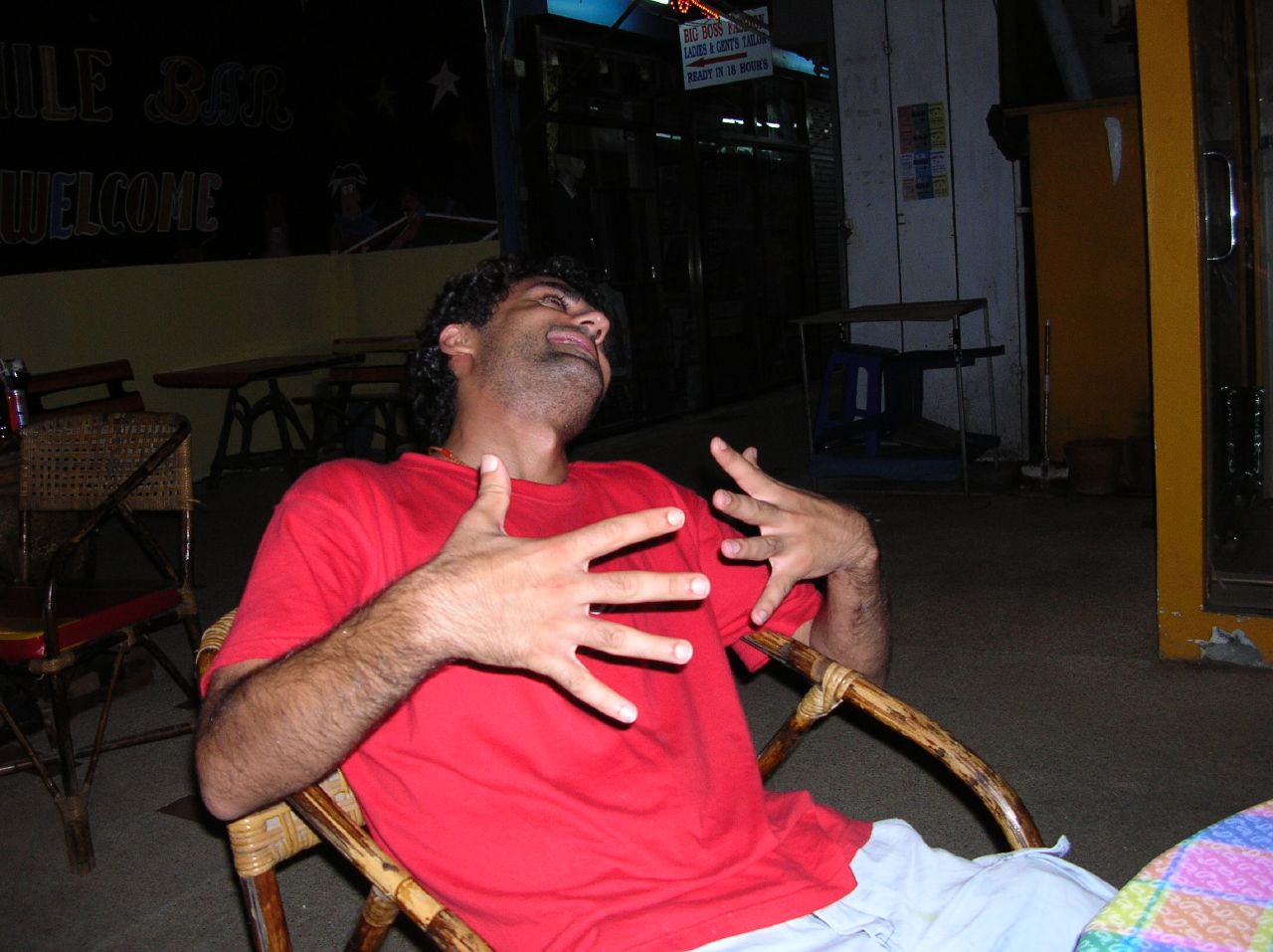This is a photograph of a man seated in a rattan or bamboo chair with curved arms and a woven backrest. He is leaning back with his head tilted to the back and right, partially obscured so only one eye, one nostril, and one ear are visible. He has dark curly hair and a five o'clock shadow, with a bit of a beard and mustache stubble. The man is wearing a red t-shirt and loose-fitting shorts, possibly khaki. His hands are raised in front of his chest with fingers splayed apart, as if mid-gesture. In the bottom right corner of the image, there is a round table with a colorful checkered tablecloth featuring pink, blue, orange, yellow, green, and purple dotted spaces. The lighting highlights his torso while his head remains more in shadow. The background reveals additional wooden and wicker chairs, tables, and a black wall structure. There are signs suggesting this may be a restaurant or bar, with the word "welcome" visible on the left side backdrop, and to the right, a small table and cabinet near a door.